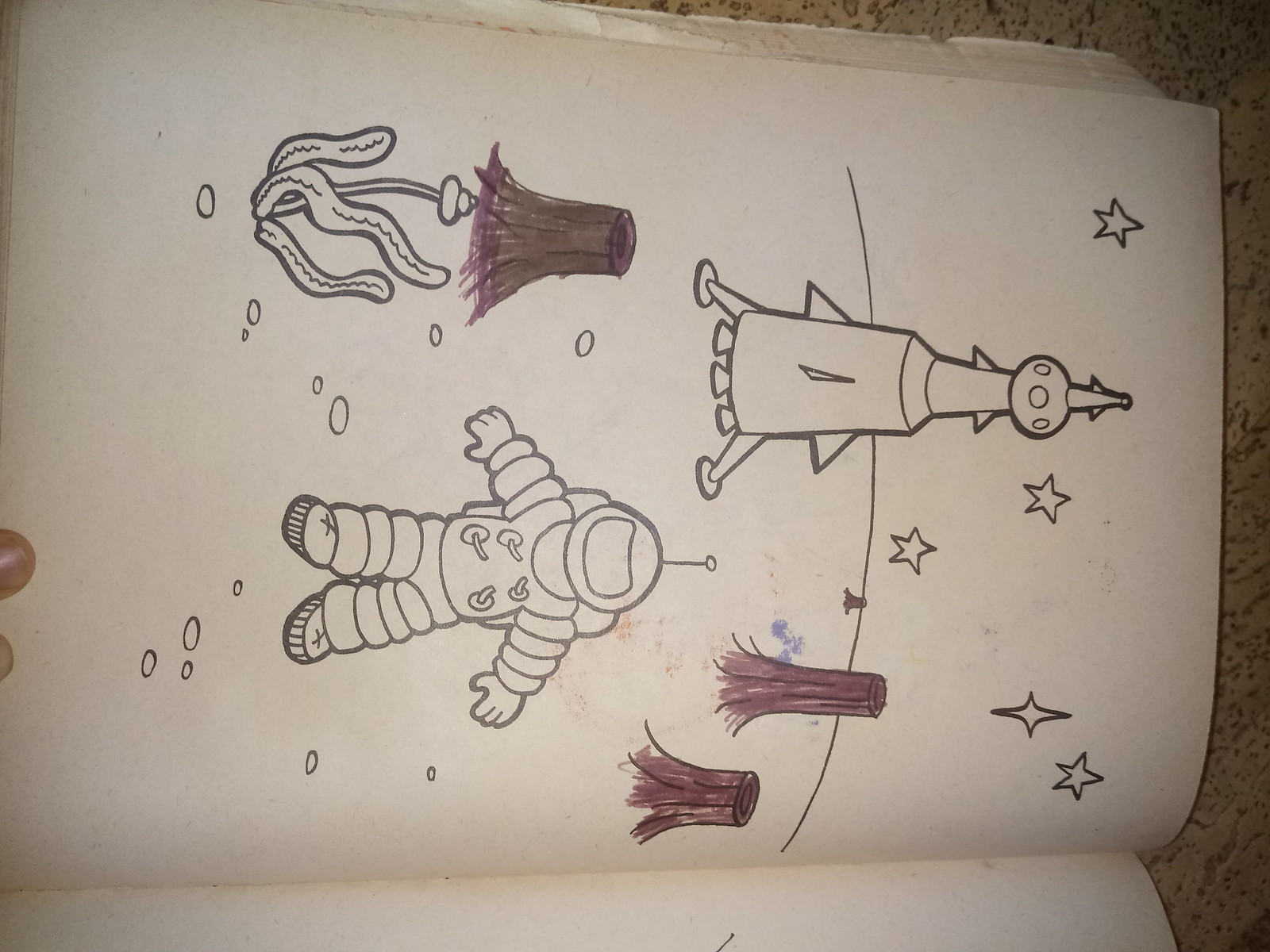The sideways-rotated left page of a child's coloring book features a rudimentary black outlined rocket ship at the center, uncolored but clearly depicted with two feet at its base, a circular section above, and a pointed top. Surrounding the rocket at the top right are several black outlined stars ready to be colored. Scattered across the page are various tree stumps; two on the right-hand side, partially colored in brown, and another on the top left side colored in brown and purple. Beneath this tree stump is a wavy long leaf stem plant. Centrally located on the page is an astronaut, portrayed in a classic space suit with a round helmet, an antenna, and a large glass visor, reminiscent of the Michelin Man. The scene also includes small craters and circles dotted throughout, adding to the space-themed motif. The top right corner of the image reveals a beige and brown countertop, indicating that the coloring book page is held open, partially visible is the tip of someone's finger.